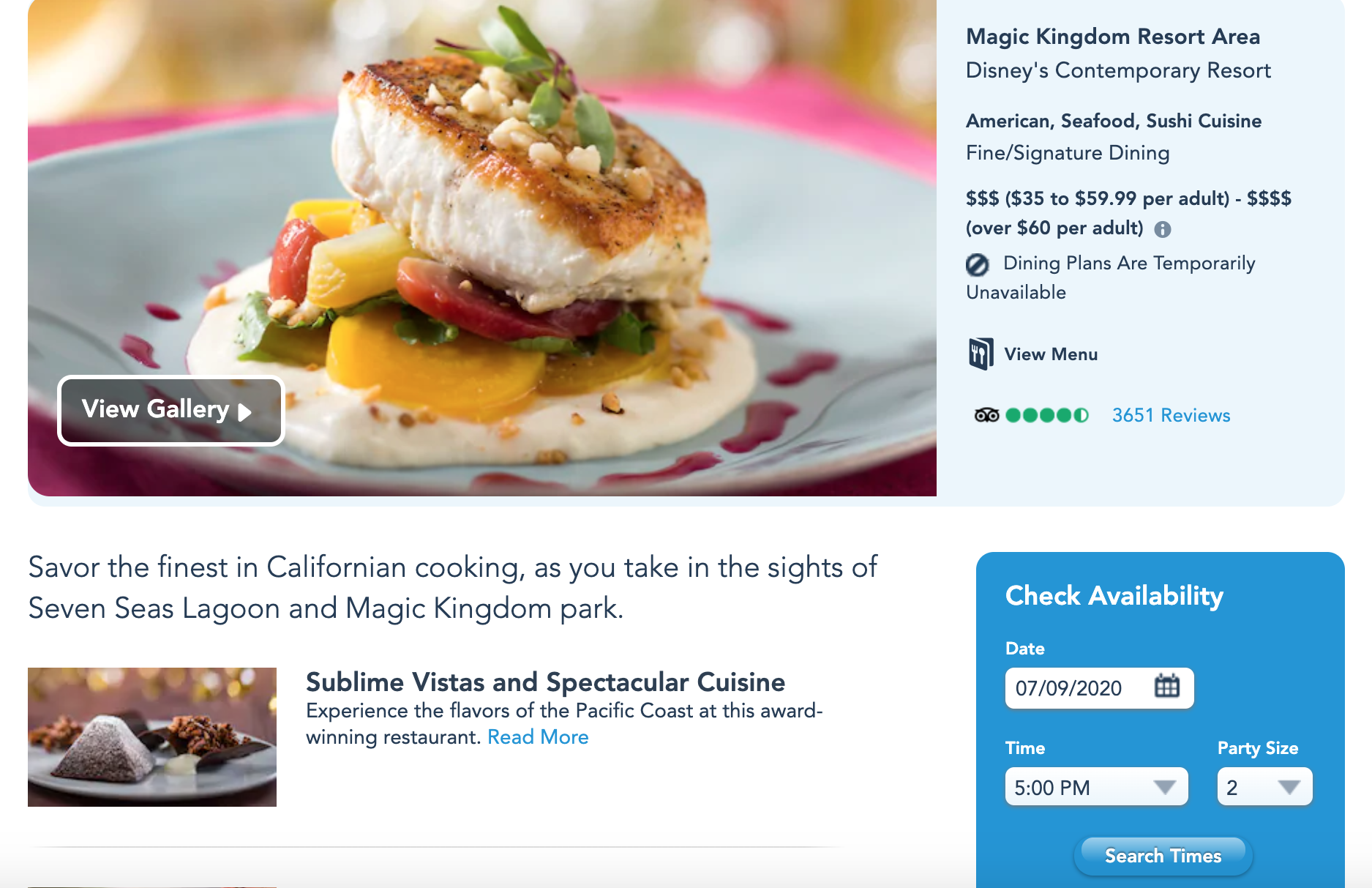The image showcases a webpage for Disney's Contemporary Resort dining options, specifically highlighting an American Seafood Sushi Cuisine restaurant. The description on the right side is in dark blue text on a light grey background, providing details about the dining experience:

- Location: Magic Kingdom Resort Area
- Venue: Disney's Contemporary Resort
- Cuisine: American Seafood Sushi
- Dining Style: Fine or Signature Dining
- Price Range: $35-59.99 per adult, with options over $60 per adult
- Note: Dining plans are temporarily unavailable
- Reviews: 3651 reviews are indicated in blue text, with green dots representing a 4.5-star rating on TripAdvisor, accompanied by the TripAdvisor logo.

On the left side of the webpage, there's an appetizing image of sushi, featuring white and yellow pieces topped with green leaves, red tomatoes, fries, and a pink sauce, all presented on a white plate. Below this image is a light black button labeled "View Gallery."

The bottom section of the background is white and includes the following text, also in blue:

- "Savor the Finest in California Cooking as you take in the sights of Seven Seas Lagoon and Magic Kingdom Park."
- "Sublime Fiestas and Spectacular Cuisine: Experience the flavor of the Pacific Coast at this award-winning restaurant."

Additionally, there's a blue section on the right side with a "Check Availability" panel that allows users to select a date, time, and party size. Below these options is a blue "Search Times" button.